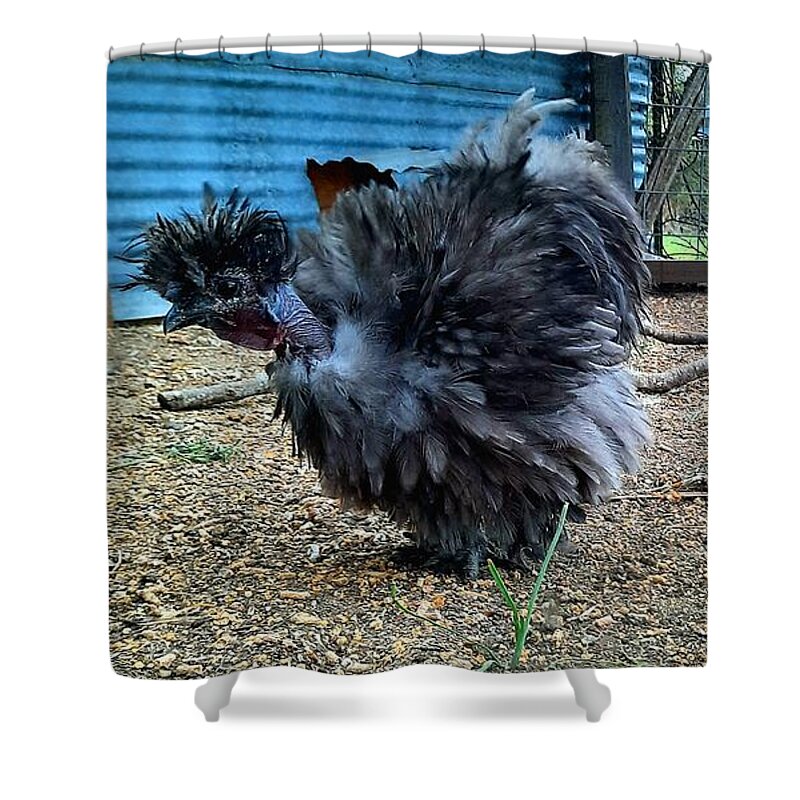In the image, a small, fluffy bird, resembling a rooster and adorned with an abundance of feathers, stands on a dirt and gravel floor. The bird, primarily gray with some black and white feathers, has a distinctive feature of long black feathers on its head that create a mohawk-like appearance. The setting includes scattered bits of twigs, leaves, and sparse blades of grass dotting the ground. Behind the bird, a corrugated blue metal sheet forms part of a pen-like enclosure, complemented by horizontal bars and chicken wire. The background also features a tree and additional branches, adding to the natural outdoor environment. The bird's fluffy and feathery demeanor stands out, making it an exotic and captivating subject against its rustic surroundings.